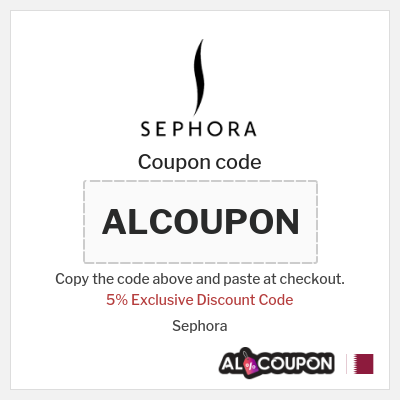A screenshot featuring a promotional banner on a white background with a gray border. At the center, the recognizable black "S" logo of Sephora is prominently displayed. Below the logo, there's a gray rectangle containing the coupon code "AL". Instructions are provided, stating: "Copy the code above and paste at checkout" to avail a 5% discount. The text is highlighted in red for emphasis. Additionally, there is an illustration of a clothing tag which is purple at the bottom and red at the top, adorned with a percent symbol on the right. The word "coupon" is written clearly on the tag. In the bottom-right corner of the image, there is a small square in a red/burgundy shade.